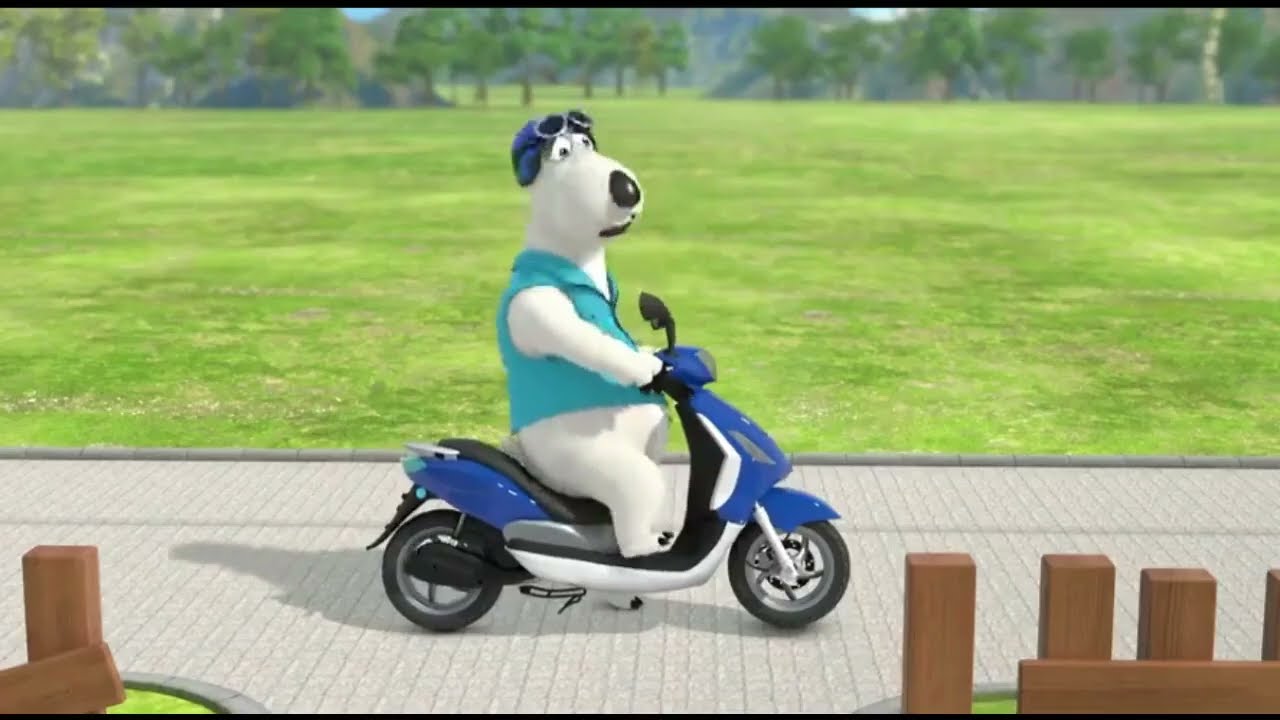The image depicts a scene from an animation or cartoon featuring a white dog, possibly a bear, riding a blue and white electric scooter. The dog is outfitted in a light baby blue vest, a blue helmet, and goggles that rest above its eyes. It appears stationary with one foot on the concrete ground, casting a shadow. The animal's expression suggests worry or concern. Surrounding the main subject, the scene encompasses a paved area lined with dark gray concrete, bordered by brown wooden slats on either side. In the background, there is a large grassy field leading to scattered trees and distant mountains, under a glimpse of sky. The color palette includes shades of blue, white, gray, brown, yellow, and green.